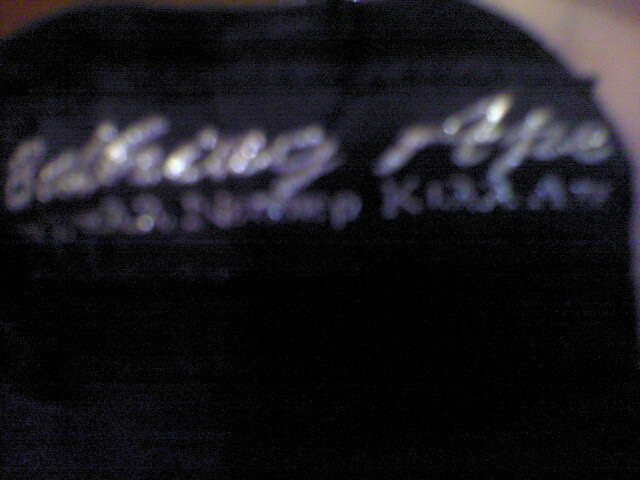In the image, we see a very close-up and blurry photograph of what seems to be a black hat, possibly a beanie, with a noticeable rounded shape toward the top corners. The low resolution and grain introduce a static-like effect, particularly in the bottom left corner, complicating the clarity. On the front of the hat, faint and blurred writing in a handwritten script is visible, having a silver or white hue. The text appears to state "Bathing Ape" in silver, with additional, less discernible text below it. The background, seen only in a small portion of the upper right corner, is light tan. Despite its indistinction, the contrast between the black fabric and the silver lettering is apparent.